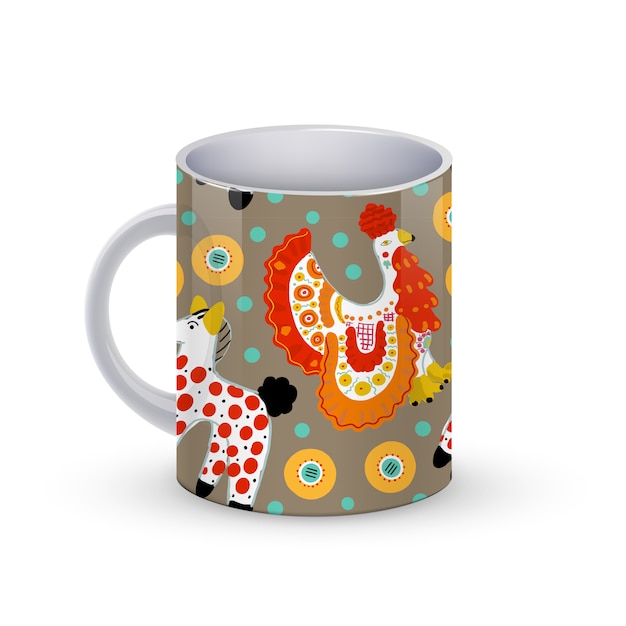This is a detailed photographic image of a ceramic mug, shown against a white background. The mug features a white handle positioned on the left side of the image and has a white interior. The main color of the mug is a grayish khaki. The design is vibrant and playful, showcasing various animals and decorative elements.

Prominently featured on the mug is a stylized white rooster. The rooster has a striking red tail, a red comb on the bottom, and a white comb on top. Its beak is yellow with a black tip, and its feet are yellow with black tips, possibly resembling toenails. Decorative elements include orange and yellow circles, blue dots, a red grid pattern on its side, and a series of check marks across its body.

Adjacent to the rooster on the left side of the mug is a white llama or horse figure, adorned with red polka dots, a black tail, yellow ears, and black stripes on its crown. Its black feet are visible, as well as a single eye shown in profile.

Additionally, the mug is adorned with various colorful circles: green circles, orange circles with blue centers, yellow circles with green interiors, and black lines encircling them. These circles are scattered across the mug's surface, with some of them partially visible as they wrap around to the other side.

Overall, the mug's design is intricate, featuring a whimsical collection of animals and geometric patterns, creating a striking and eye-catching piece.